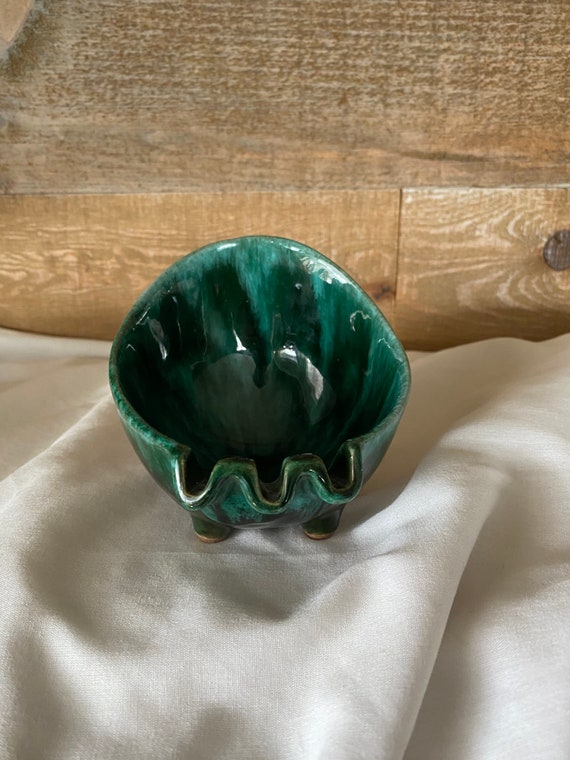This photo showcases a small, handmade ceramic ashtray, bowl-shaped and thoughtfully designed to resemble a cup. The ashtray features three small, U-shaped slots on the near side, ideal for holding cigarettes, and is distinctively higher on the far side. Painted in varying shades of glossy emerald and teal green, this piece stands out with its charming, four-legged base. The ashtray is small enough to fit comfortably in one's palm, exuding a rustic, artisan appeal. It rests on a slightly folded, beige-white linen cloth, capturing the essence of natural light, possibly from windows with curtains. The background enhances its organic aesthetic, consisting of an untreated, rough wooden wall with visible wood grains, adding a touch of rustic charm to the scene.